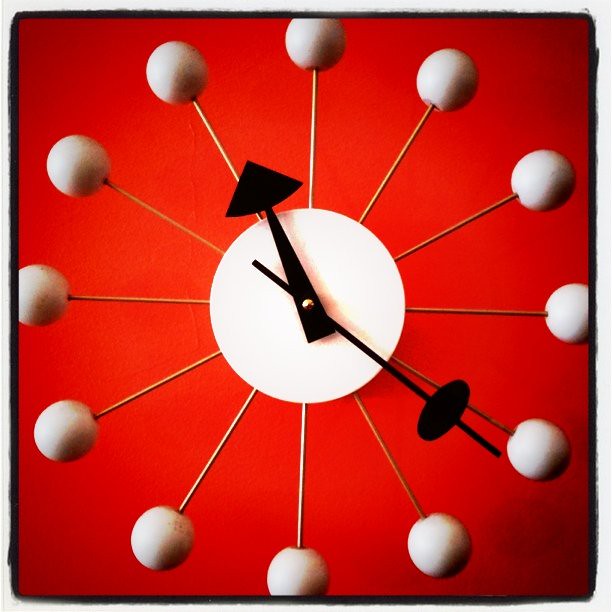A striking square clock dominates the entire frame with its bold design. Encased in a sleek black border, the clock face is primarily a vibrant red, accented with subtle black shading in the bottom right and upper right corners. At the heart of the clock is a large, pristine white circle, which houses a smaller, shiny gold circle at its center, anchoring the clock hands. The hands are a stark black, with the hour hand distinguished by a thick black triangle at its end. Uniquely, the hour hand also features a circular disc that nearly extends to its tip. Instead of traditional numbers, time is marked by white ping-pong ball-like spheres, each stationed at the end of delicate silver metal rods radiating from the outer edge of the inner white circle. The overall design is modern and geometric, combining vibrant colors with minimalist elements for a visually compelling timepiece.